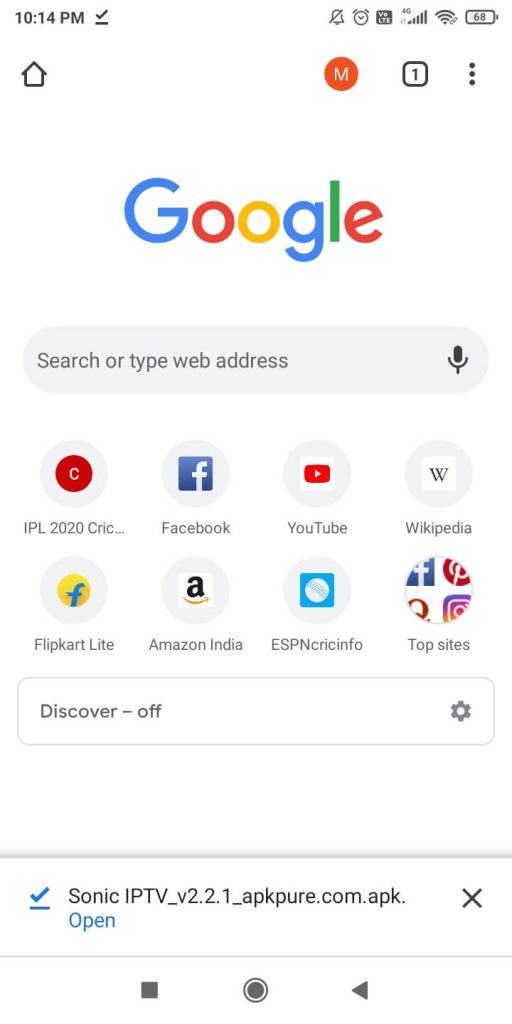This screenshot, taken on a person's cell phone at 10:14 PM, showcases various icons and details from the device's screen. 

#### **Top Bar:**
- **Time:** 10:14 PM
- **Icons (from left to right):** 
  - Bell icon with a slash (notifications muted)
  - Alarm clock icon 
  - 4G coverage indicator
  - Wi-Fi icon
  - Battery icon at 68%

#### **Below the Top Bar:**
- **Icons:** 
  - Black house icon
  - Red circle with a white "M" in the center
  - Black square with a number "1"
  - Three vertically aligned dots

#### **Google Section:**
- **Google Logo:** 
  - Letters in blue, red, yellow, blue, green, and red
- **Search Bar:** 
  - Placeholder text: "Search or type web address"
  - Microphone icon on the right side

#### **Underneath the Search Bar:**
- **Icons with Labels:**
  1. **IPL 2020 CRIC...**
     - Icon: White circle with a red circle and a white "C" in the center
  2. **Facebook**
     - Icon: Blue square with a white lowercase "f" to the right side
  3. **YouTube**
     - Icon: White square with a red rectangle in the center and a white arrow pointing to the right
  4. **Wikipedia**
     - Icon: White square with a black capital "W"
  5. **Flipkart Lite**
     - Icon: Yellow circle with a blue lowercase "f"
  6. **Amazon India**
     - Icon: Lowercase "a" with a yellow smile underneath
  7. **ESPN CRIC Info**
     - Icon: Blue square with a white circle in the center

#### **Additional Sections:**
- **Top Sites:** 
  - Icons for Facebook, Pinterest, Instagram, and a red "Q"
- **Discover Off:** 
  - Blue check mark

#### **At the Very Bottom:**
- **Text:** 
  - "Sonic IPTV_V2.2.1_APKpure.com.apk, open"

This detailed caption provides a comprehensive description of the screenshot, outlining the various icons, labels, and elements present on the screen, along with their colors and placements.